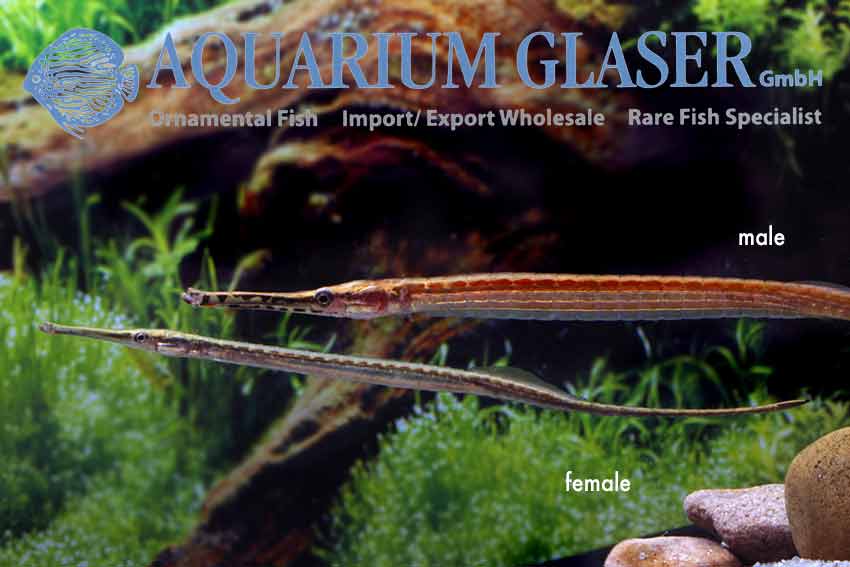The image is an advertisement banner for Aquarium Glaser GmbH, specialists in ornamental fish import/export wholesale and rare fish. The photo prominently features two needle-like fish with extremely elongated, thin bodies and long, pointed heads. One is labeled "male" in white text and is orange-red in color, while the other, labeled "female," is smaller, thinner, and light green. The fish appear to be in a tank that contains rocks in the bottom right corner, faux green vegetation both at the top and bottom, and a wooden stump in the background. At the top of the image, large blue text reads "Aquarium Glaser," accompanied by a blue fish logo, and below, smaller gray text describes their specialization.